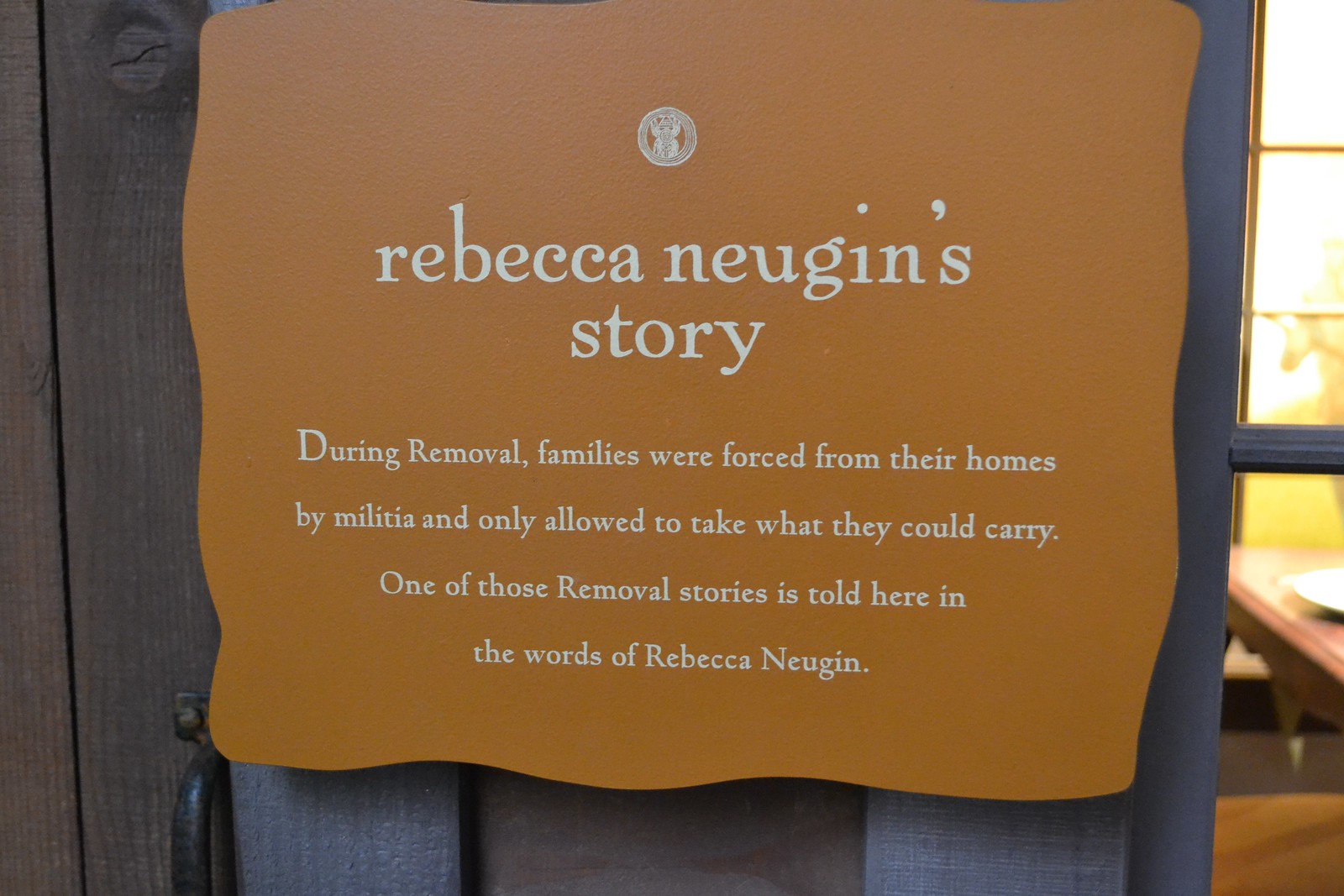This photograph is a close-up view of a brownish-orange plaque with slightly curved edges, hanging on a wooden wall next to a door with vertical wooden boards and a black, rusty handle located towards the bottom left of the image. The plaque features a small, artsy white logo at the top that is difficult to make out clearly. Below the logo, in large white letters, it reads "Rebecca Nugent's Story," with the following text in smaller white letters: "During removal, families were forced from their homes by militia and only allowed to take what they could carry. One of those removal stories is told here in the words of Rebecca Nugent." The right side of the image reveals a bluish-gray windowpane through which a charming interior is visible, including an elegant table, sunlight streaming in through another window, and nice wooden floors. The setting juxtaposes the somber message of the plaque with the warmth and charm of the interior space.